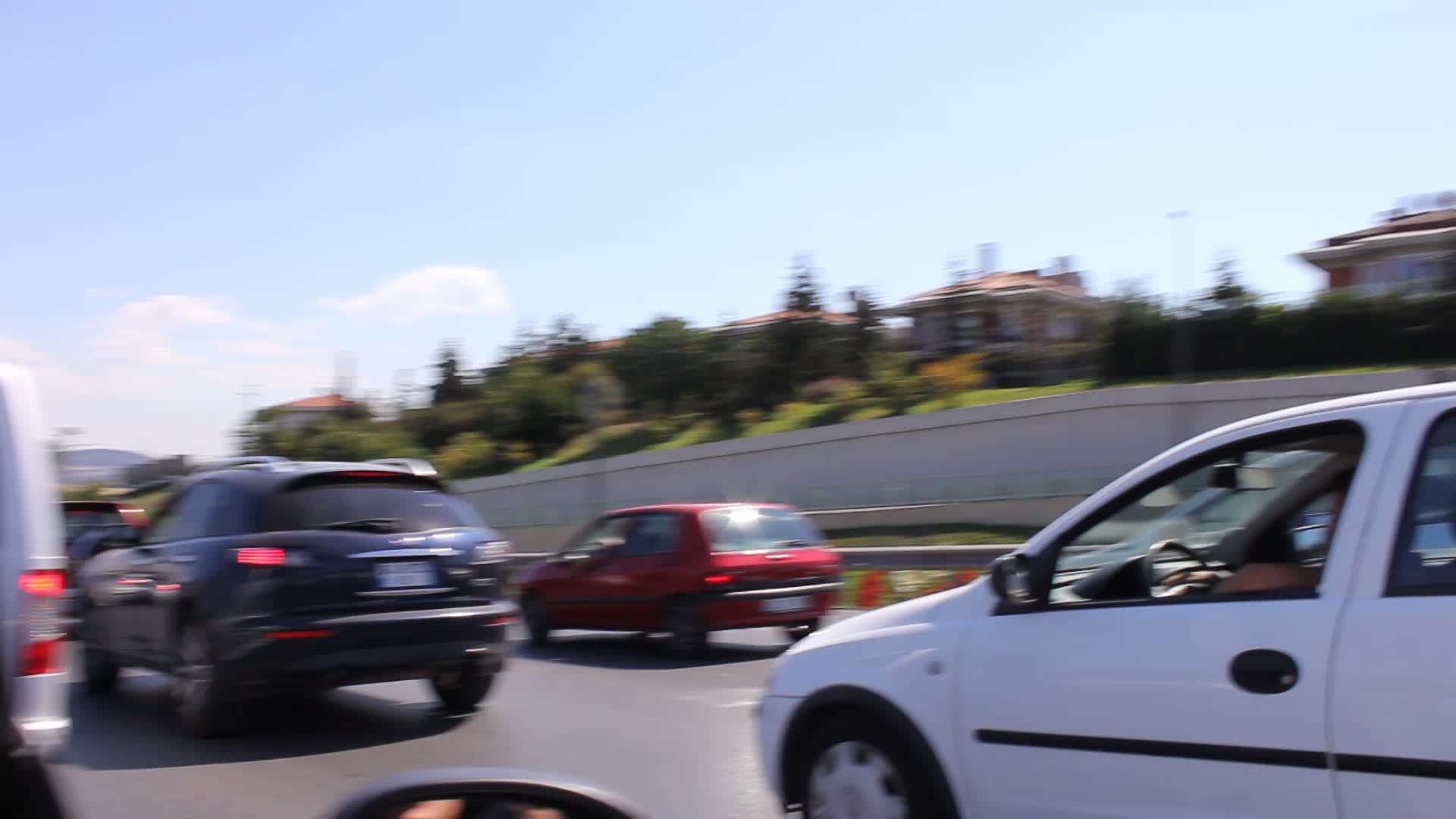This image captures a bustling scene on a freeway, likely taken from the passenger side of a moving vehicle. The foreground prominently features a white car immediately to the right with a visible driver behind the steering wheel. Ahead of this vehicle, there is a bluish-black SUV, while a white van-like vehicle can be seen to its left. To the right of the SUV is a red, slightly boxy compact car. In the background, a stone wall edges the freeway, with a lush green hillside above it. The hill is dotted with grass, trees, and distant houses. The sky above is a soft blue with scattered clouds, and a glimpse of colorful flowers lines the side of the street, adding a touch of nature to the urban landscape.